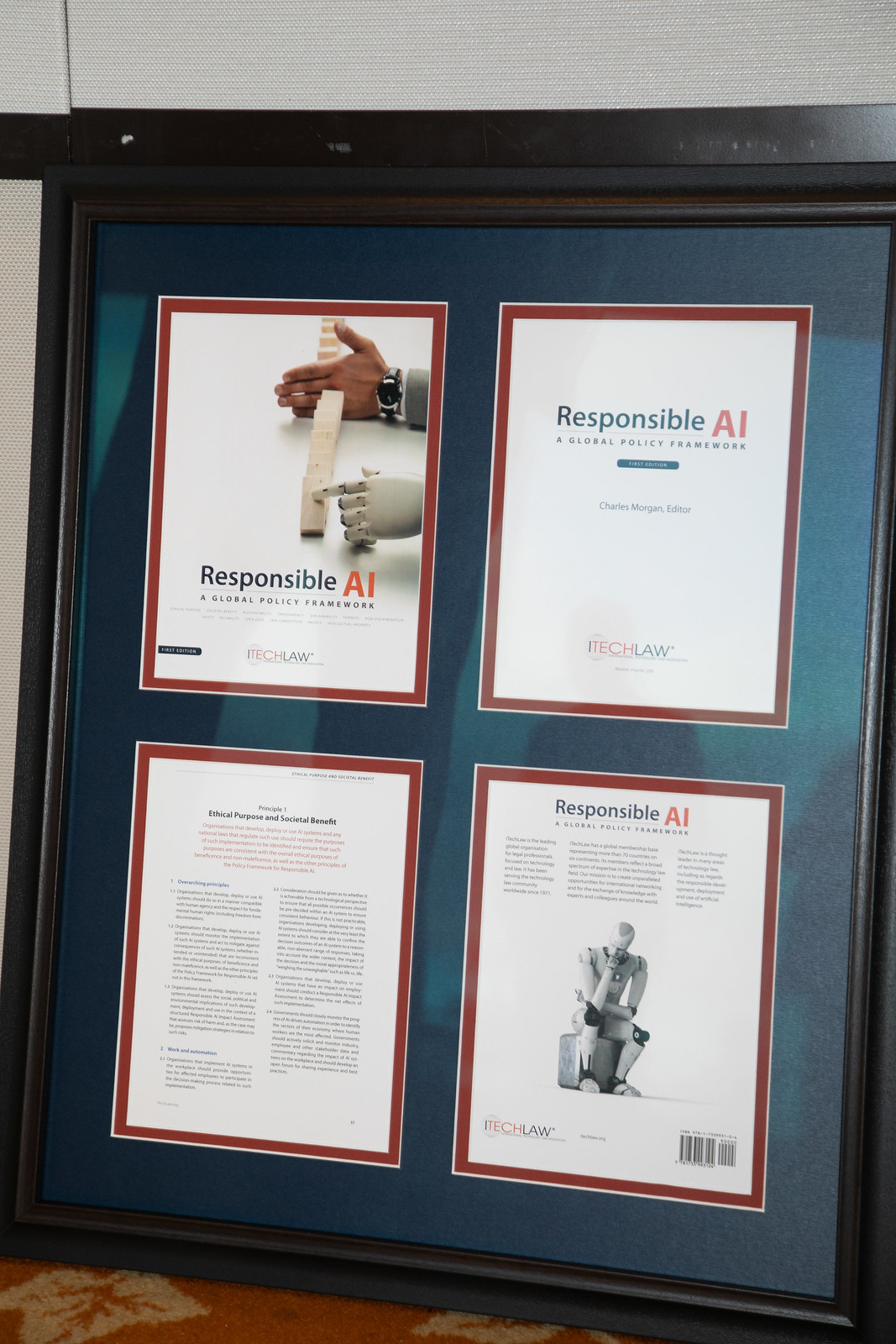The photograph inside a convention center or hotel features a framed sign resting on an orange carpet with a beige leaf print pattern, against a white wall. The dark blue-framed sign has a dark teal background divided into four sections, each with a red border and white paper. 

In the top left section, "Responsible AI" is inscribed above an image depicting a robot hand and a human hand coming together. The top right section displays the title "Responsible AI, a Global Policy Framework" and mentions "iTech Law." 

The bottom left section contains two columns of small, unreadable text. However, it includes a title, "Principle 1, Ethical Purpose and Societal Benefit," hinting at detailed principles or policies governing AI technology. 

The bottom right section shows a robot in a thinker pose, sitting on a stool or rock, with a barcode placed in the bottom right corner. The text above echoes the theme with "Responsible AI, Global Policy Framework."